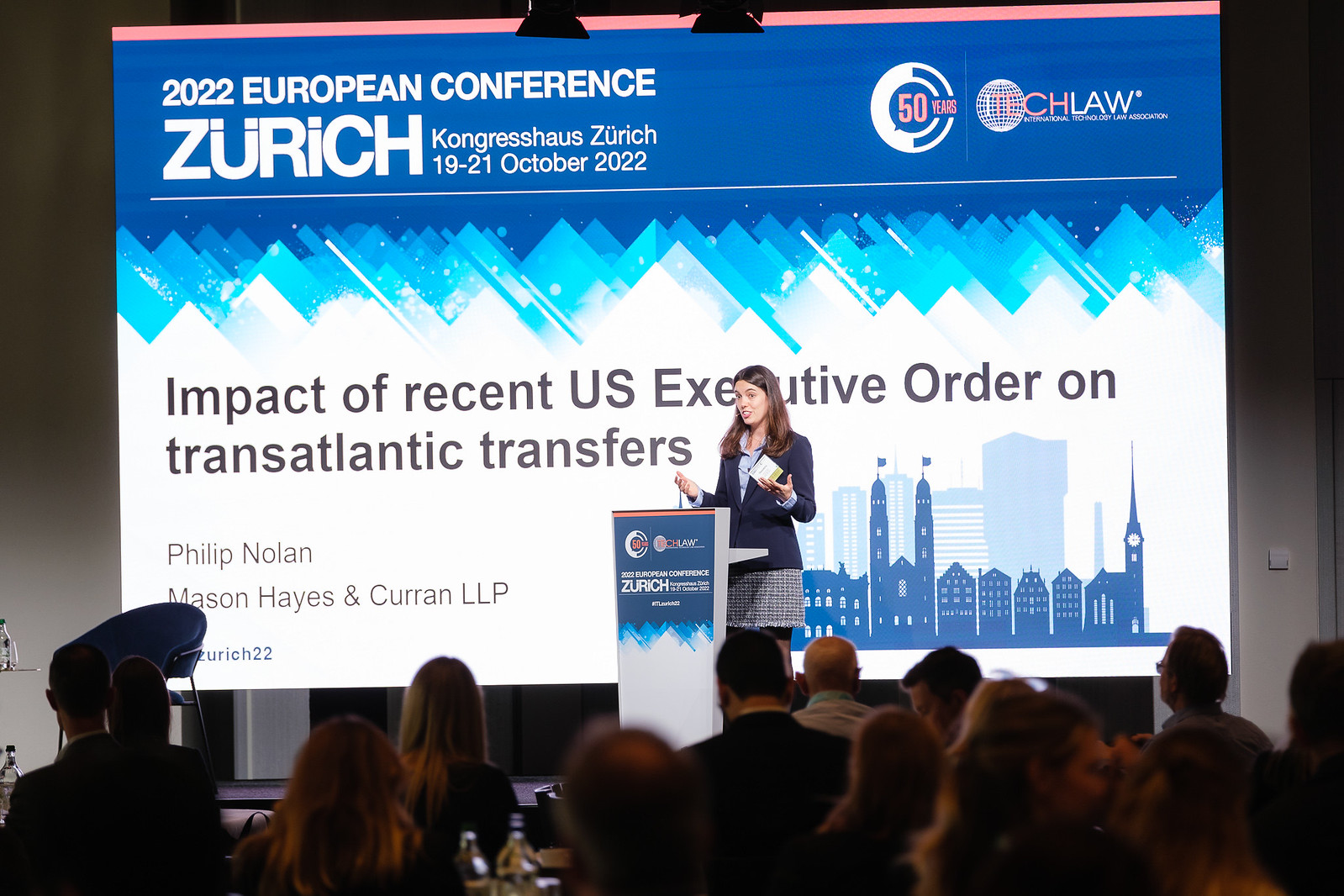In the image, a woman with long brown hair is standing at a podium on a stage, delivering a presentation. She is dressed in a blue blazer, a light blue shirt, and what appears to be a gray skirt or pants. The podium features the logo of the Zurich conference, matching the large screen behind her. The screen prominently displays "2022 European Conference, Zurich, Congress House, Zurich, 19-21 October 2022" in blue and white text. The central text on the screen reads, "Impact of recent U.S. executive order on transatlantic transfers," and a logo reading "50 CH law" is visible on the right side. Additionally, the screen includes text such as "Philip Nolan Mason, Hayes, and Curran LLP." The setting is indoors, and shadows of the heads of the audience members are visible in the foreground, signifying that she is addressing a crowd at this conference. The room is filled with varying shades of gray, black, brown, silver, white, light blue, dark blue, and orange, contributing to the professional and serious atmosphere of the event.